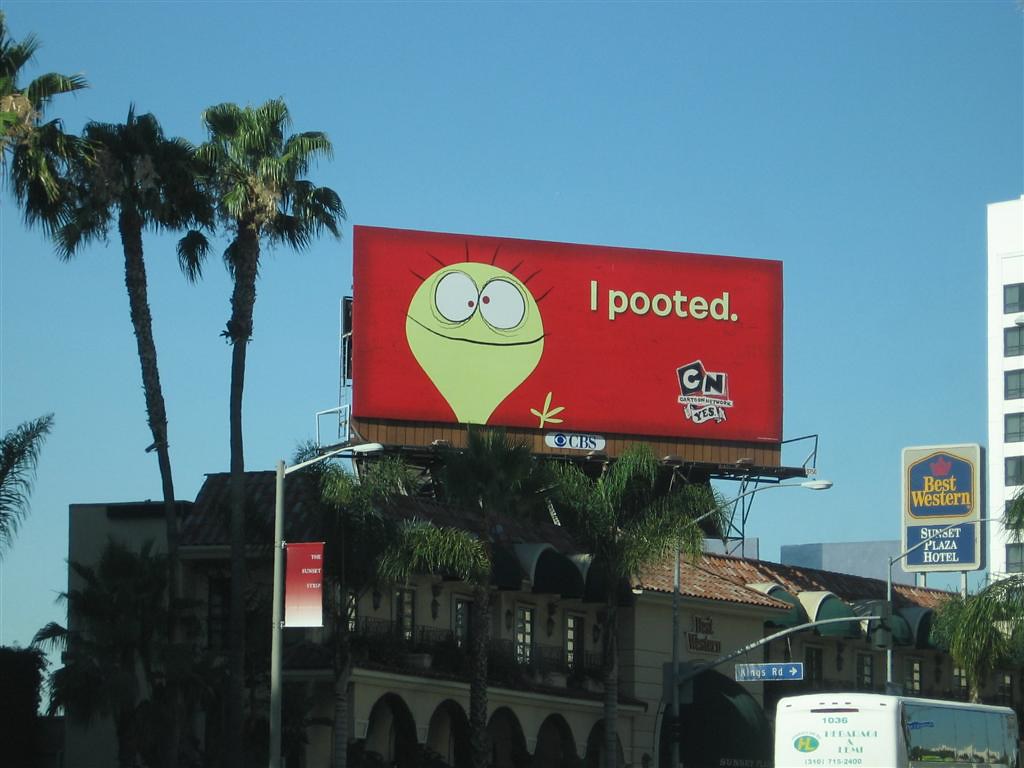This vivid photograph captures the dynamic urban scene of a bright sunny day, featuring a striking red billboard above a hotel building in what appears to be a bustling city area, likely in California. The hotel building, identifiable as the Best Western Sunset Plaza Hotel, is a two-story structure with a Spanish-style roof and charming little balconies. Tall palm trees tower around the building, with smaller ones in front, adding a tropical touch to the urban landscape. Adjacent to the hotel, a blue sign with white text pointing to Kings Road stands prominently, indicating the street name.

The centerpiece of the image is the vibrant red billboard promoting Cartoon Network. The billboard features a whimsical green alien character with an almost hot air balloon-shaped head. Its face is quite expressive, with a huge horizontal smile that nearly bisects it. The alien's eyes are large, round, and cross-eyed with bright red pupils, giving it a quirky look. The character also sports spindly hair lines, a raised left hand with four fingers, and the catchphrase "I pooted" written beside it in the same light green color. Below this text, the familiar Cartoon Network logo is displayed in black and white blocks, with a slightly crooked 'C'. In the background, the clear blue sky adds a vivid contrast to the scene, further illuminated by a partial view of a white tall building with at least seven visible floors, and a possible hotel shuttle bus captured near the bottom right of the image.